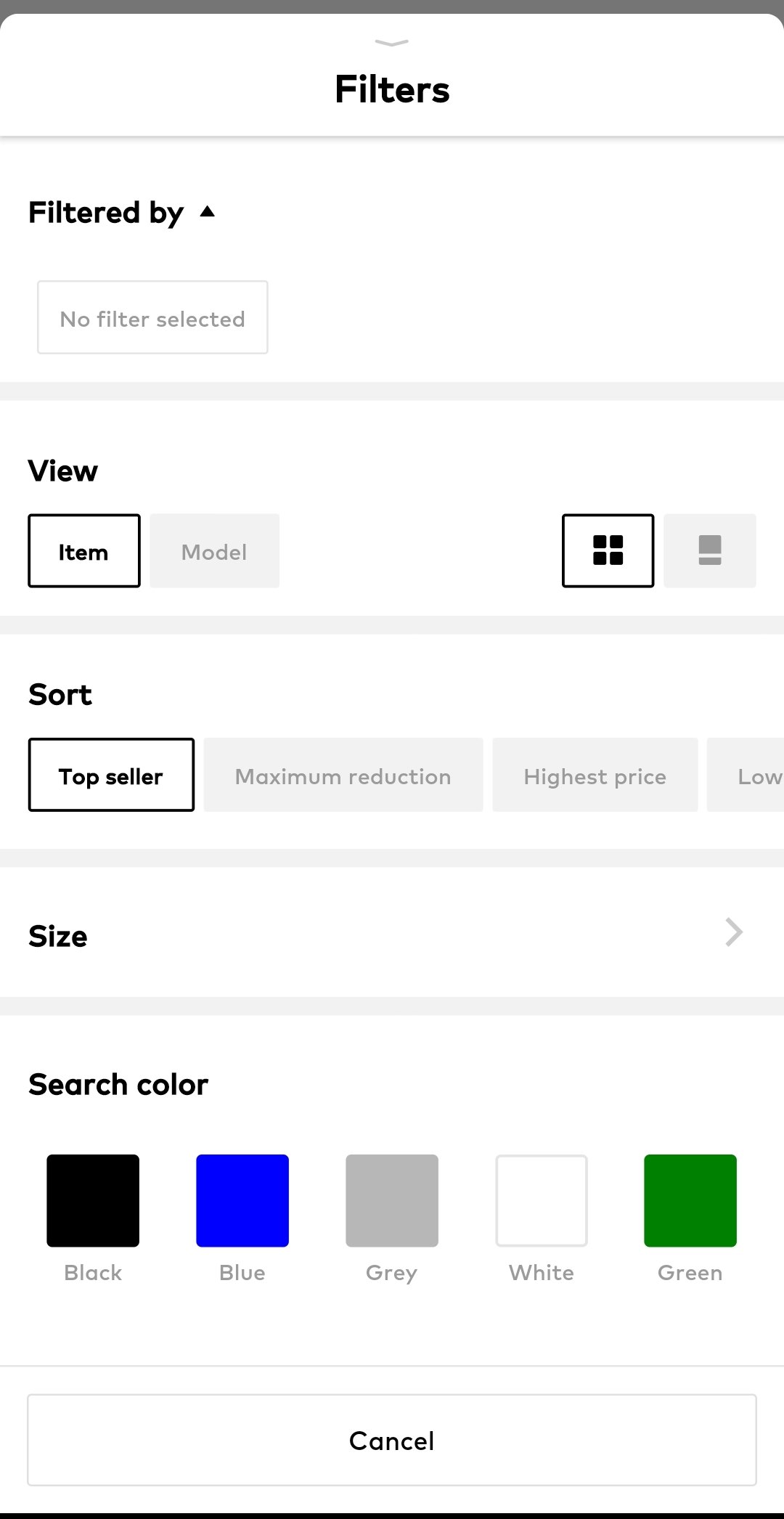The image showcases a screenshot of a filter page from a mobile application, most likely on an Android device. At the very top and centered, the title "Filters" is displayed. The page is divided into four distinct sections for users to customize their search experience.

1. **Filter By:** The first section titled "Filter By" currently has no options selected.
   
2. **View:** The second section, labeled "View," offers two modes - "Item" and "Model." The user has chosen the "Item" mode.
   
3. **Sort:** The third section, named "Sort," shows that the user has opted for the "Top Seller" sorting choice. To the right, other available options include "Maximum Reduction," "Highest Price," and "Lowest Price."
   
4. **Search Color:** The final section at the bottom is "Search Color," which allows users to filter by specific colors such as black, blue, gray, white, and green.

A "Cancel" button is positioned at the very bottom center of the screen. The background of the page is predominantly white, providing a clean and simple interface.

This page serves as a filter tool for refining search results within a website or application, offering customization through views, sorting options, and color selections.